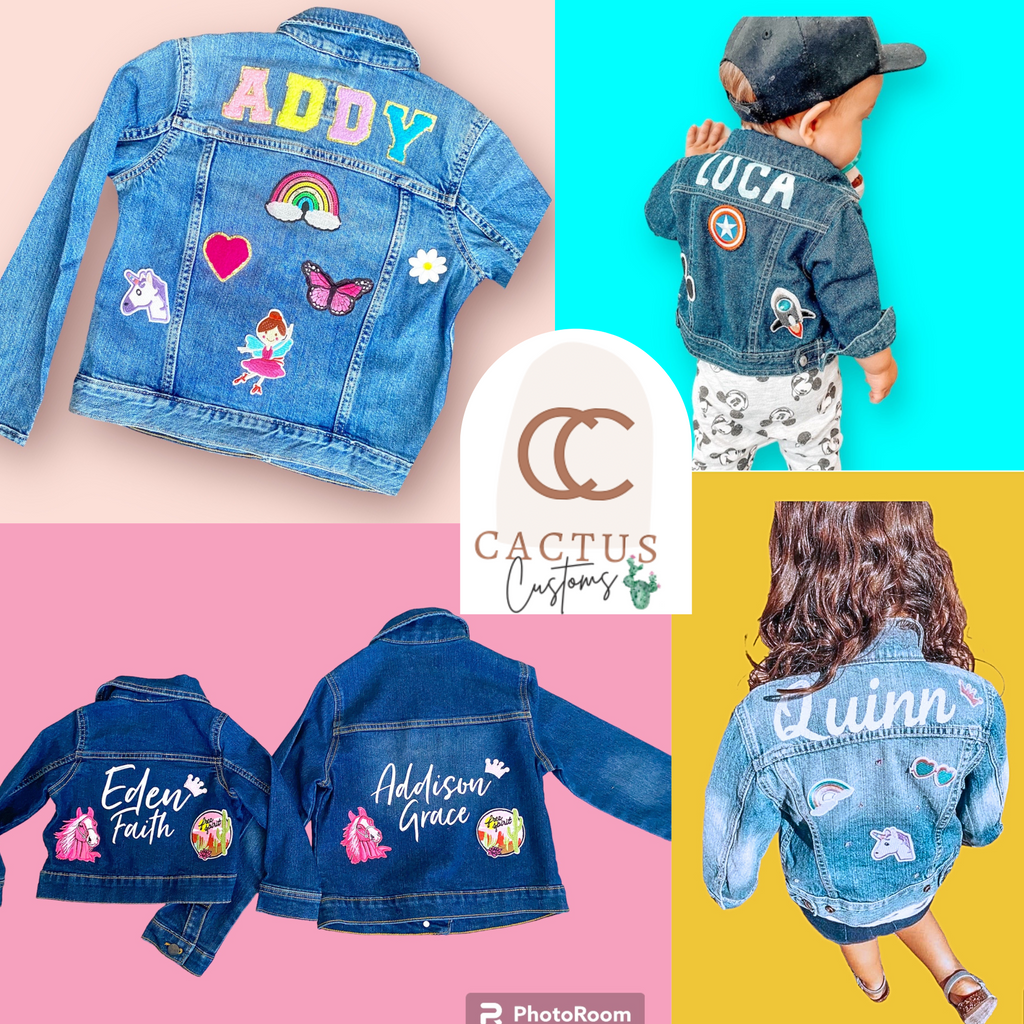This advertisement for Cactus Customs features a logo with two overlapping C's at the center, encircled by four square images showcasing personalized denim jackets for children. The top left panel displays a light blue jean jacket with “Addie” in colorful patches. Below “Addie” are various vibrant patches: a unicorn, a pink heart with a gold outline, a rainbow ending in clouds, a pink and purple butterfly, a cute ballerina fairy, and a daisy. The top right panel features a toddler in a dark blue denim jacket with “Luca” painted on the back along with patches of a star and a rocket ship, against a teal background. The bottom left panel shows two dark denim jackets labeled “Eden Faith” and “Addison Grace,” each adorned with patches depicting a horse and a desert scene with cacti, set against a pink background. The bottom right panel presents another child with long brown hair, wearing a light blue denim jacket labeled “Quinn” in cursive, decorated with patches of a unicorn, rainbow, hearts, and a crown, set against a yellow background. Together, these images showcase the customization options available at Cactus Customs, allowing customers to personalize denim jackets for children with names and various colorful patches.